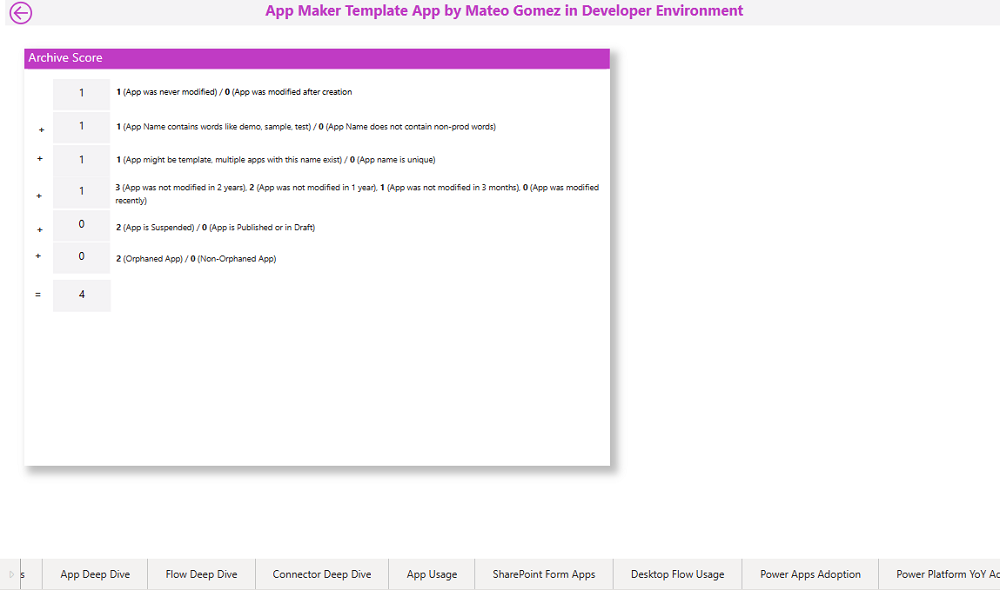**Caption:**

The image showcases a detailed launch page for a website or web app, primarily related to application management and analysis. Over the top 5% of the image, a light gray bar features a back arrow icon in purple and the text, "App Maker Template App by Mateo Gomez in Developer Environment."

Below the gray bar, a prominent purple banner with white text reads, "Archive Score." To the left, a gray number input box is available for keying in numbers. Adjacent to this box is a vertical list of app-related criteria and scores including:
1. App was never modified.
2. App was modified after creation.
3. App name contains words like Demo, Sample, Test.
4. App name does not contain non-grad words.
5. App might be a template.
6. Multiple apps with this name exist.
7. App name is unique.
8. App was not modified in 2 years.
9. App was not modified in 1 year.
10. App was not modified in 3 months.
11. App was modified recently.
12. App is suspended.
13. App is published or in draft.
14. Orphaned app.
15. Non-orphaned app.

Each criterion is accompanied by scores or selectable options.

At the bottom of the image, a gray menu bar with black lettering features various navigation options, specifically: App Deep Dive, Flow Deep Dive, Connector Deep Dive, App Usage, SharePoint Forum Apps, Desktop Flow Usage, Power Apps Adoption, and Power Platform Year-Over-Year (YOY).